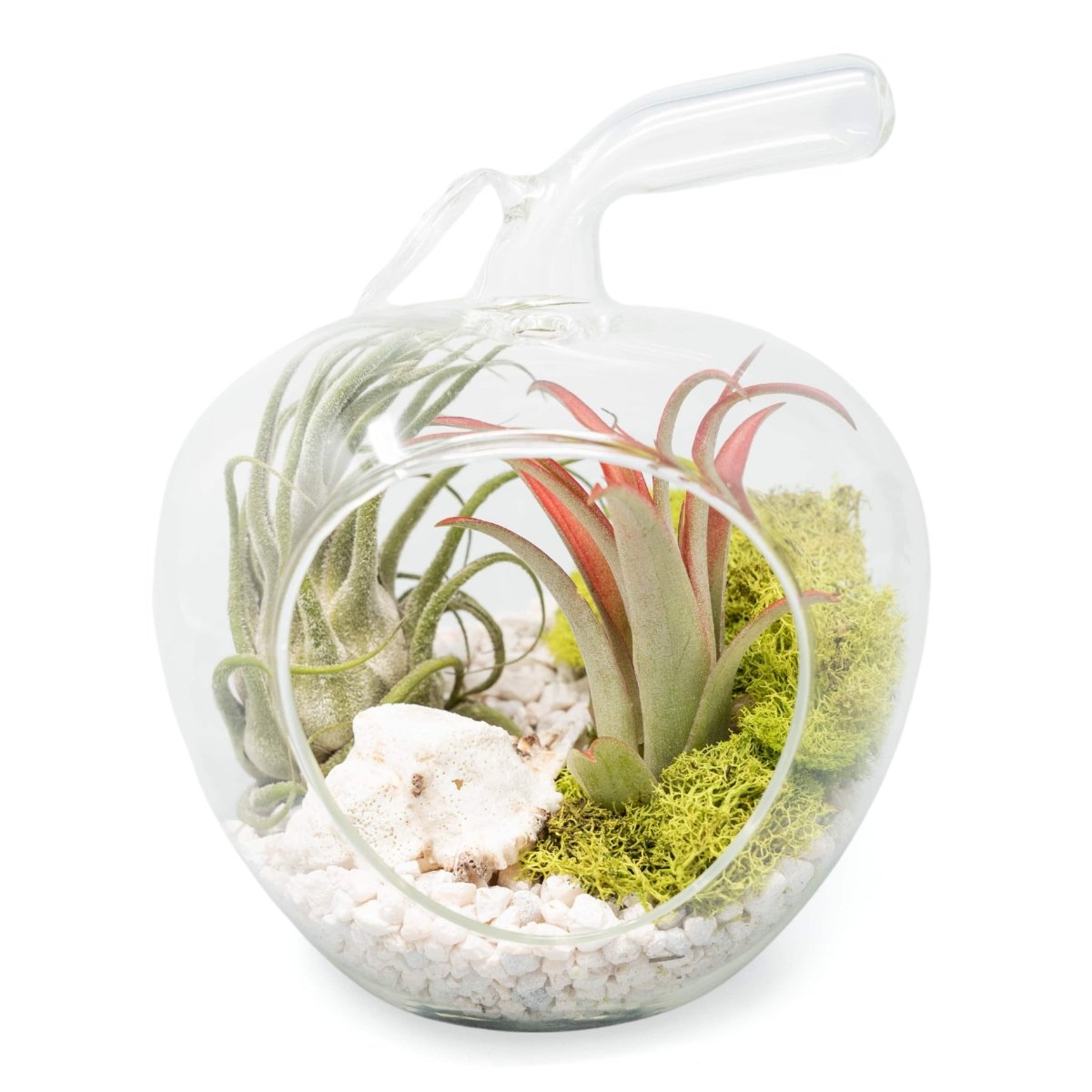This image showcases a delicate terrarium housed inside a clear, apple-shaped glass container. The container features a rounded body with a small, clear glass stem protruding from the top, complemented by a clear glass leaf. The apple's front displays an opening through which the lush interior is visible. Within the glass confines lie several elements: there are grayish-white pebbles on the bottom, along with two distinct plants. The plant on the right has green and pink spiky leaves, adding a striking contrast, while the one on the left has slender stalks with tapered points and green bulbs. Interspersed with these plants is a feathery, fern-like greenery. Additionally, green moss wraps around the right plant, contributing to the miniature garden's vibrant ecosystem. The overall setting suggests an indoor environment, as the glass terrarium presents a controlled, decorative habitat for the plants.